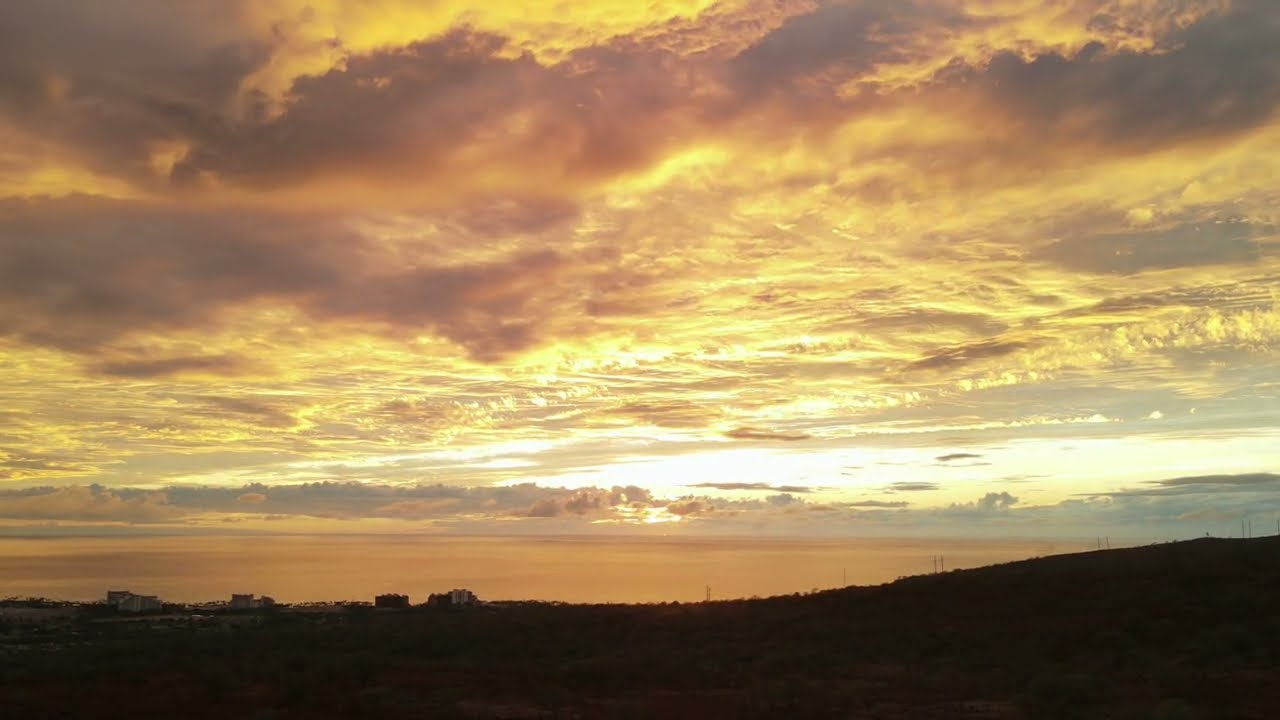This photograph captures an enchanting outdoor scene during either sunset or sunrise. The majority of the ground at the bottom of the image is dark and covered with grass or small plants, and it appears dim due to the low light conditions. On the left edge of the ground, there are obscure small buildings or settlements, possibly houses or industrial structures, that are difficult to precisely identify. The sky, which is the standout feature of the photo, is a mesmerizing tapestry of clouds in various hues – dark green, golden, orange, yellow, pink, and light blue. These clouds form a compelling pattern against the backdrop of a softly illuminated sky, creating a serene and picturesque vista. On the horizon, a hill and power lines can be discerned, adding depth to the composition. The mixture of colors in the sky, paired with the dark foreground, gives the entire scene a striking contrast and a tranquil, almost magical ambiance.